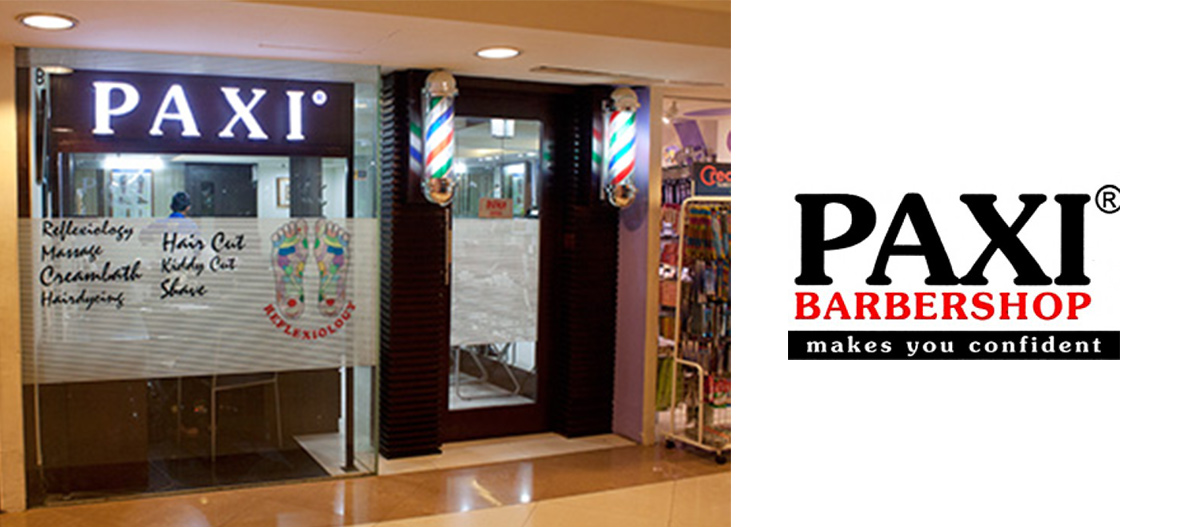A detailed front view of the Paxi salon, located in an indoor mall, showcasing its black-framed entrance door flanked by iconic cylindrical barber lights adorned with red, white, and blue slanted stripes. The upper section of the frontage prominently displays the Paxi logo in white on a black rectangular background. Below the logo, there's a lit-up sign surrounded by a transparent section that transitions into a light gray banner with the inscriptions: "Reflexology, Massage, Cream Bath, Haircut, Kid Cut, Shave," in clear text. The expansive floor-to-ceiling windows, alongside the door, feature a white band across the midsection that offers partial privacy while hinting at the services inside. To the right of the window, an image depicting two feet highlights the reflexology services. The vibrant, colorful lights at the top of each side of the entrance enhance the inviting atmosphere of this modern barbershop and salon.